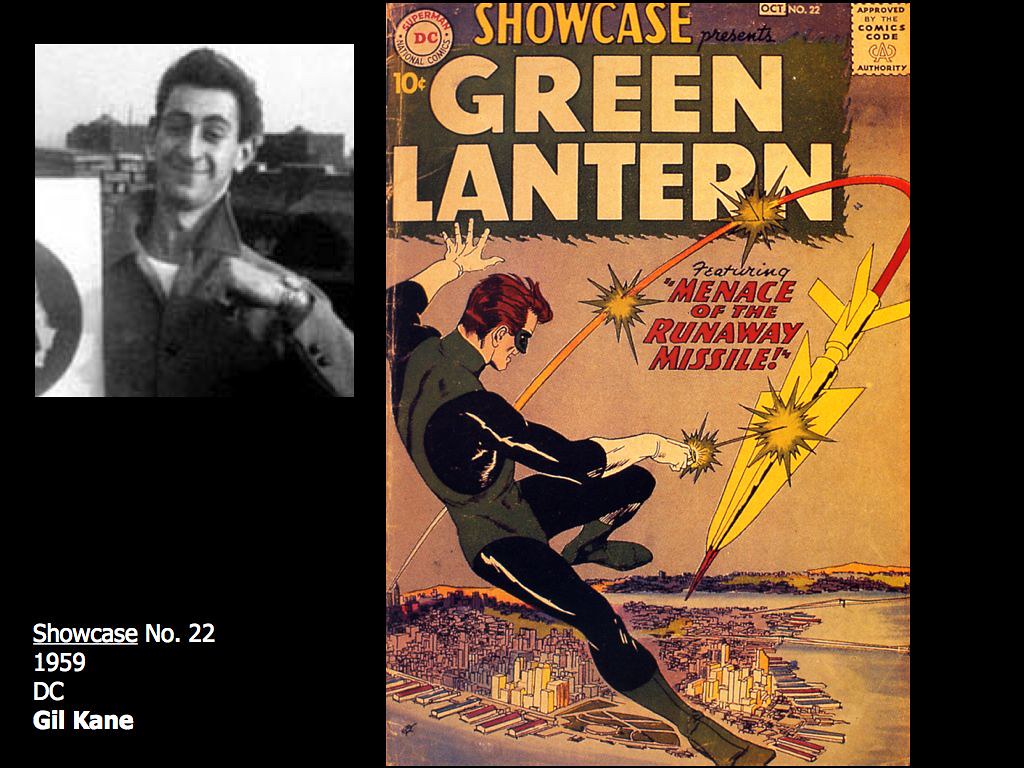The image is split into two segments, each providing a rich context of a vintage comic book and its creator. On the left, there's an older black-and-white photo of a man in his 30s with neatly styled hair, dressed in a collared shirt with the collar slightly popped. He is smiling at the camera. Below his photo, the text reads "Showcase No. 22, 1959, D.C., Gil Kane." This identifies the man as Gil Kane, a notable figure associated with the comic.

To the right of his photo is the cover of a Green Lantern comic book. The cover headline reads "Showcase Presents," with "Green Lantern" prominently displayed in bold white letters. The issue is marked as number 22, from October 1959, and was priced at 10 cents according to the insignia on the top left-hand corner. The artwork on the cover features the Green Lantern character dressed in a black and green suit—complete with a mask and distinct red hair—confronting a yellow missile that appears to be targeting a city. In red ink, the cover also features the caption "Menace of the Runaway Missile," highlighting the thrilling storyline within.